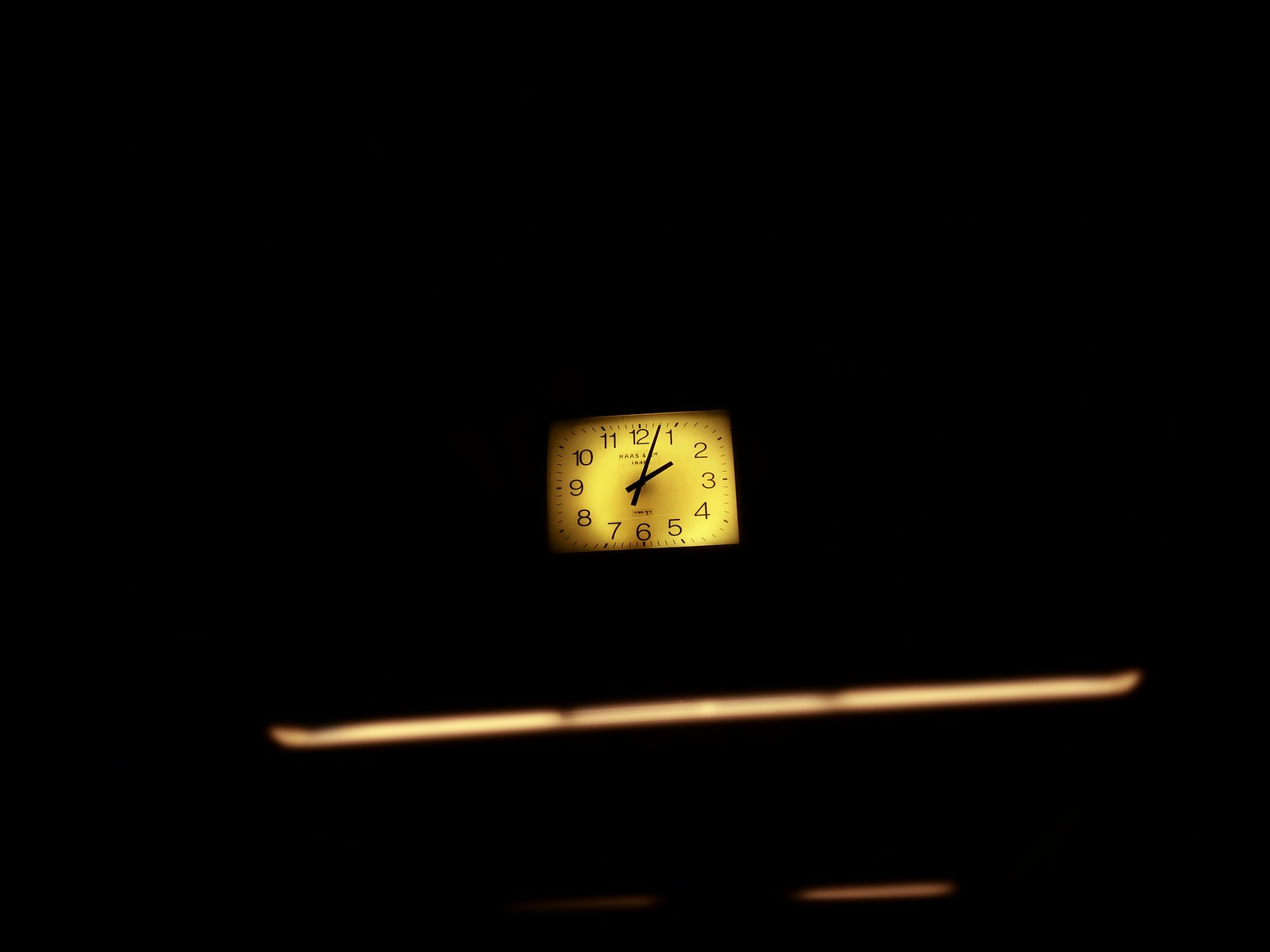The image is a dark, color photograph taken in what seems to be a night setting, as it is almost entirely pitch black. At the center, the focal point is a square-shaped analog clock with a face that emits a golden-yellow glow, suggesting the presence of a backlight. The face of the clock is a warm, golden yellow, with black numbers from 1 to 12 arranged in a traditional clock format. The clock hands indicate the time is approximately 1:03. Below the clock, there is a glowing rod or line that arches slightly upward at both ends, with an orangey glow, and a smaller sliver or line of light beneath it, in a darker orange hue. The rest of the image is completely immersed in darkness, heightening the luminous elements of the clock and the lines below it.